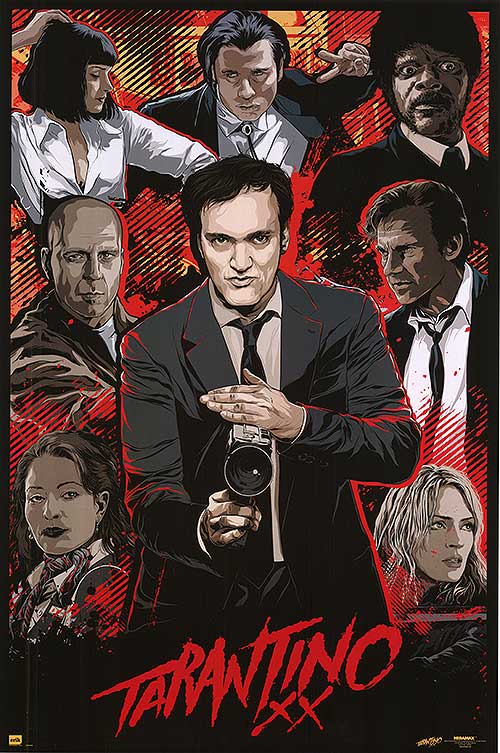This image is a visually-striking, digital or hand-drawn painting featuring Quentin Tarantino surrounded by characters from his iconic film **Pulp Fiction**. Dominating the center, Tarantino is attired in a dark gray suit, light gray shirt, and black tie, holding a camera in front of his chest. His right hand's splayed fingers partially obscure the camera. The surrounding characters, rendered in a cartoonish style with adept use of light and shadow, bolster the composition's dramatic effect.

At the bottom left, a woman with dark brown hair and a brown coat looks directly forward. Above her, a bald man with light brown skin in a dark brown suit is depicted. To his right, a prominent woman with short black hair and an open-neck white shirt is illustrated. Directly above, another character, featuring black hair, a white shirt, and a black suit, forms a peace sign with his hand. In the upper right corner, a black man with wide eyes, an afro, and a dark suit with a white collar stands out. Below him, a man with dark brown skin and hair, wearing a loose black tie and white shirt, angles leftward. At the very bottom, a woman with almost blonde hair faces right.

The composition’s lower section bears the bold, red inscription "Tarantino" followed by two X's, suggesting an artistic signature. The entire piece adheres to a minimalist color scheme of black, white, and red, enhancing its stylized graphic appeal.